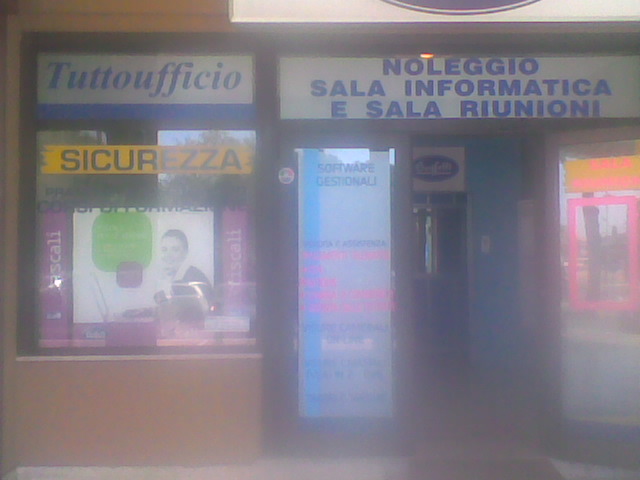The blurry photo captures an entrance to a business establishment with a storefront visible from the sidewalk. The lens appears to be fogged, lending an almost opaque, smoky appearance to the image. Prominently displayed at the top left is a white sign with blue writing, reading "TUTTO UFFICIO." Directly below it is a yellow banner stating "SICUREZZA," also in blue letters. Underneath these banners is an image of a woman looking towards the viewer, flanked by a green and a purple box to her left. This visual element is surrounded by a purple border that is difficult to decipher due to the glare and blurriness.

Toward the right and top of the storefront, another white sign with blue text reads "NOLEGGIO SALA INFORMATICA" and "ESALA RIUNIONI." The entrance door to the establishment is open, revealing blue walls inside. Above the door, there is a small white border featuring an indistinct blue oval with white writing that remains unreadable. Signs appear vibrant with various colors, predominantly blue, yellow, and black, adding to the storefront's visual appeal and seemingly advertising different services, possibly related to software or office security.